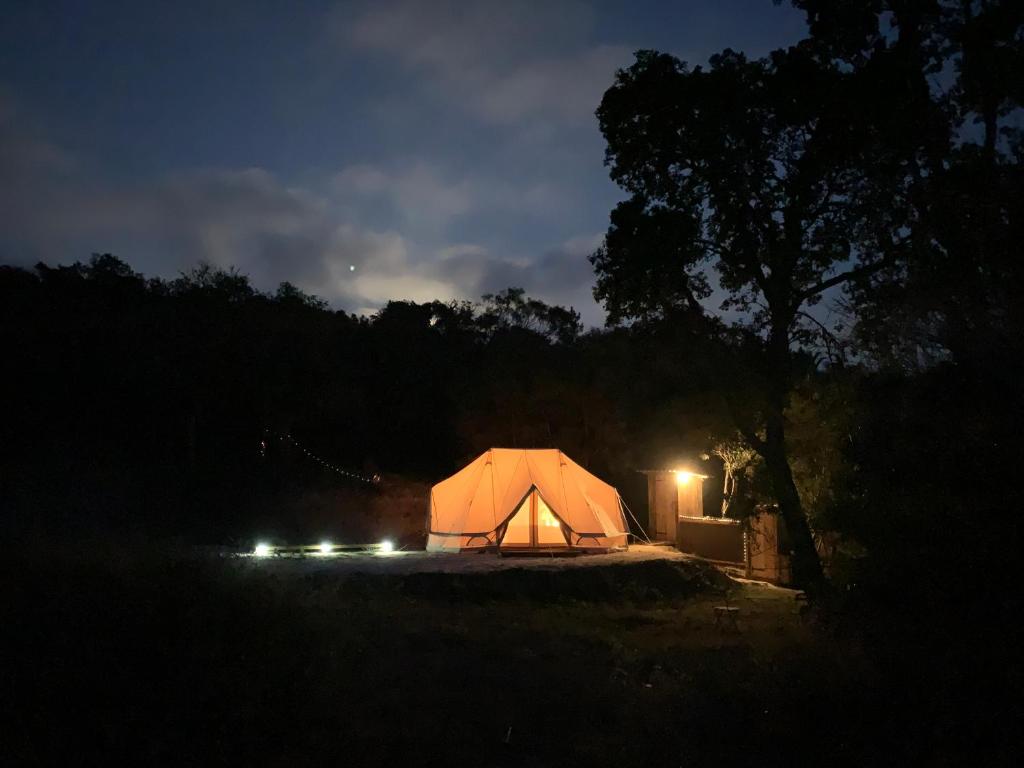In this photo, a tranquil camping scene unfolds just after sunset. The sky retains a faint blue hue, accented by patches of white clouds and possibly illuminated by moonlight. Silhouetted trees frame the campsite, indicating it is likely spring or summer, given their full foliage. The focal point is a well-lit, large tan canvas tent, clearly prepared for occupants, as evidenced by its bright illumination and level, worked-out foundation. A series of three ground lights leads up to the tent, further enhancing its visibility. Behind the tent, there appears to be a wooden outhouse with a light on its side, adding a rustic touch to the scene. In the foreground, a prominent tree stands silhouetted against the dusky sky, grounding the image in a serene, natural environment.